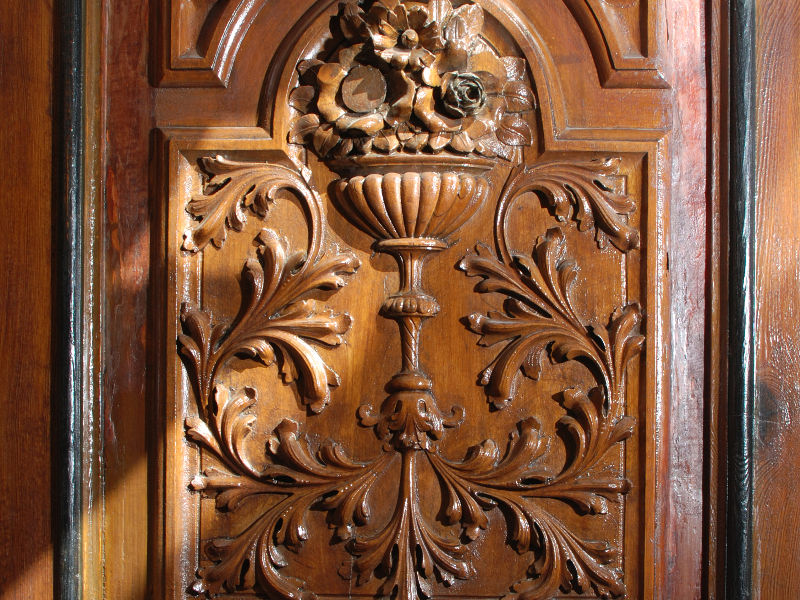This close-up photograph captures a richly ornate wooden panel, likely a door, featuring intricate carvings and a varnished, smooth surface that gleams in the sunlight. The panel, which is primarily brown and seems to resemble either maple or redwood, is bordered by darker, almost black lines framing the composition. At the top, an elaborate vase or flower pot overflows with finely detailed flowers, each distinct in appearance—possibly a daisy, a rose, and a poppy—crafted with meticulous attention to detail. These floral carvings extend outwards, accompanied by an array of long, expressive leaves, all skillfully created using a rotary tool to impart texture and depth. The woodwork's ornate design lends an old-world charm and a sense of timeless craftsmanship to the piece.